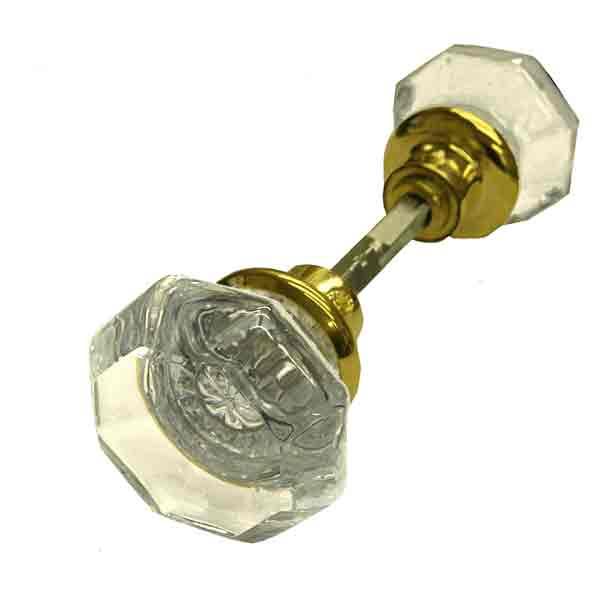The image features a vintage doorknob set that appears to be from the 1970s or 1980s. The central focus is the intricate detailing of a clear, glass-like knob contrasted by its gold mounting hardware. Both the left and right ends of the knob set are visible, showing the gold components that house the actual doorknob mechanism. A central bolt, intended to secure the doorknob assembly into a door, is positioned diagonally across the image. The visible knob on the left is angled towards the bottom left corner, while the opposing knob is oriented towards the upper right, suggesting the photo is taken from a slightly leftward perspective. The clarity of the detailing on the left knob provides a striking contrast to the obscured view of the right, enhancing the nostalgic appeal of the vintage hardware.